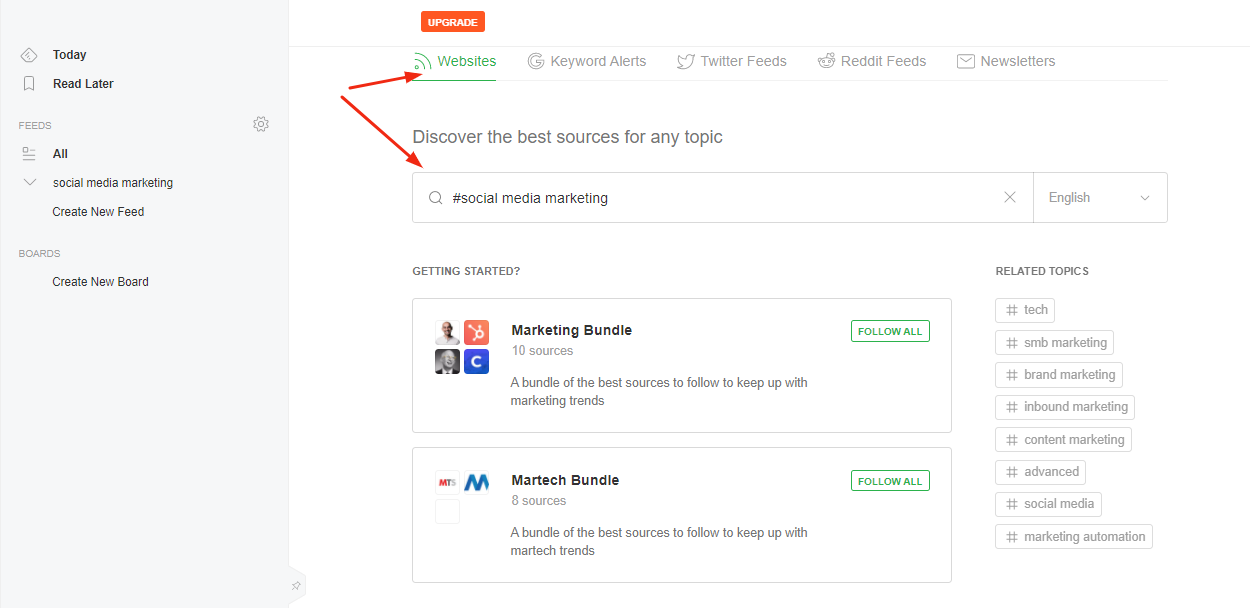This image showcases a website's browsing feature interface designed to help users discover and follow content sources. At the top of the interface, there is a prominent header with the word "Upgrade" displayed in white font on an orange background. Below this header, a navigational menu presents several options in light gray letters: "Websites," "Keywords," "Alerts," "Twitter Feeds," "Reddit Feeds," and "Newsletters." The option "Websites" is highlighted in green and indicated by two orange arrows.

Further down, text in bold type reads, "Discover the best sources for any topic." Beneath this, a search bar contains the hashtag "#SocialMediaMarketing." Next to the search bar is a small dropdown menu labeled "English."

Below the search bar, the page introduces users to different content bundles. The first bundle, labeled "Marketing Bundle," is accompanied by four small images and offers "10 sources," described succinctly with the caption, "A bundle of the best sources to follow to keep up with marketing brands." Users have the option to "Follow All" links in green.

Another section below features the "MarTech Bundle," providing "8 sources," along with a description that it includes "a bundle of the best sources to follow to keep up with marketing trends." This section also displays four placeholder boxes, with two filled in. One box features a large blue "M."

To the far left, a vertical rectangle houses various navigational links in dark black text: "Today," "Read Later," "All," "Social Media Marketing," "Create New Feed," and "Create New Board." This layout suggests an intuitive interface focusing on enabling users to efficiently access and organize their chosen content.